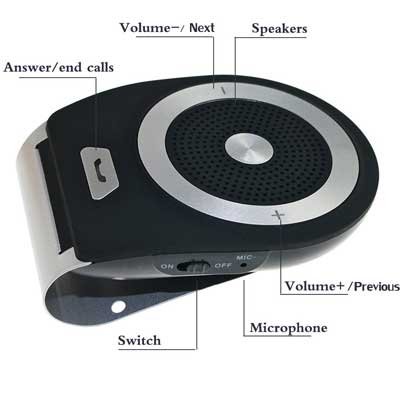This detailed image showcases an electronic speaker device, centrally positioned and taking up the entire frame. The color scheme includes black, white, silver, and gray tones. Prominently, the top of the device features a distinctive chrome circle containing a black circle, which in turn encloses a smaller chrome circle. This design element is accompanied by various buttons and labels indicative of its multifunctional capabilities. 

On the left side, a silver button with a phone symbol is designed for answering and ending calls, as indicated by the "answer/end calls" label. The front side of the speaker includes an on/off switch and a microphone input jack. Surrounding the chrome circle, there are plus and minus symbols used for volume control or navigating to the next or previous functions. Text on the screen further clarifies the functions of these controls, including "volume," "volume+/previous," "next," "speaker," "microphone," and "switch."

This well-positioned electronic device, possibly an image from an instructional manual or product website, highlights its various features and user interface components for handling calls and controlling audio playback.